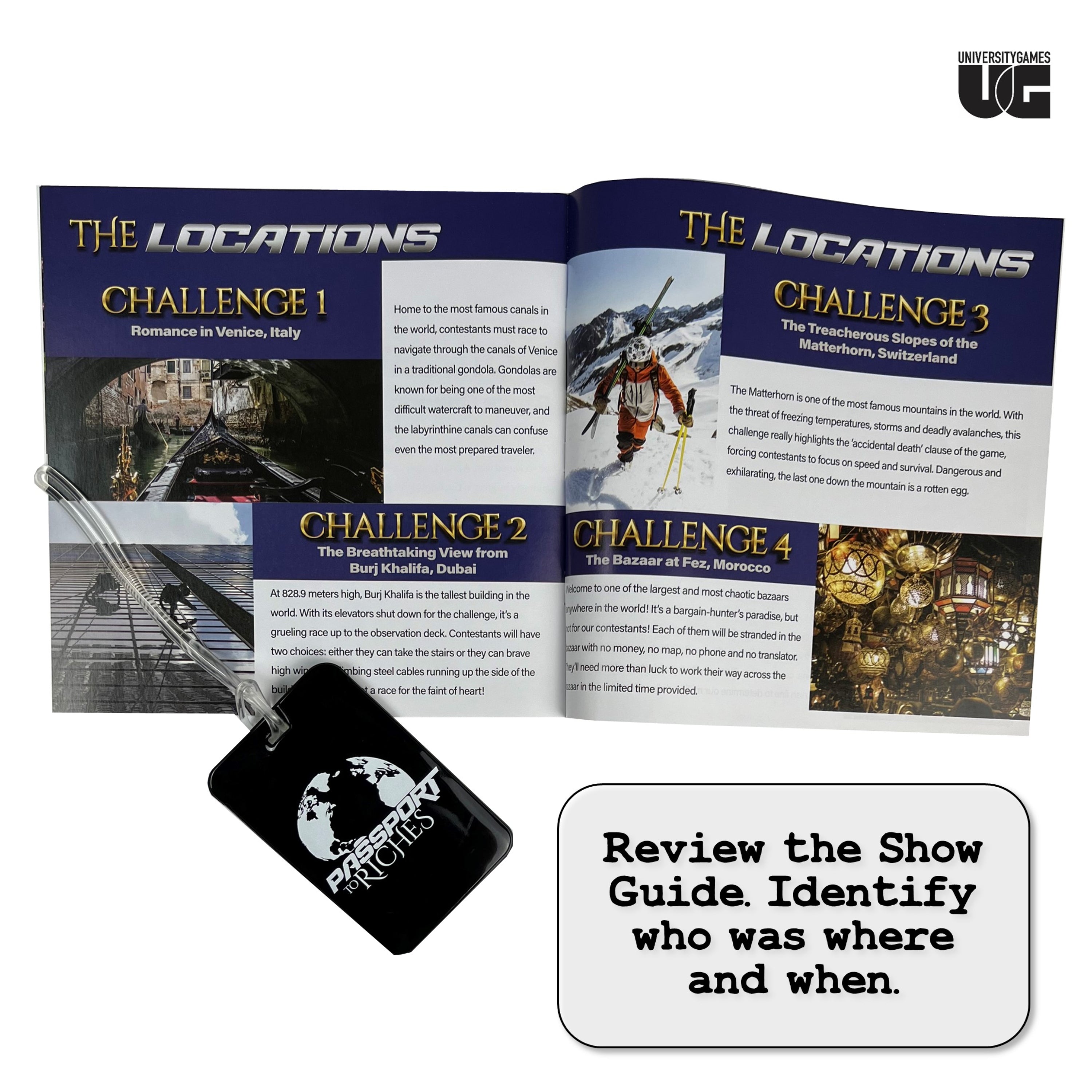In the top right corner, the image features a logo inscribed with "University Games UG." The main focus is an open magazine or brochure against a white background titled "The Locations" at the top left. The magazine reveals four detailed challenges, each accompanied by vivid images depicting the respective locations.

Challenge 1: "Romance in Venice, Italy" features a scenic image of a gondola gliding down a canal beneath a picturesque bridge, written in elegant gold lettering.

Challenge 2: "The Breathtaking View from Burj Khalifa, Dubai" showcases a dramatic upward perspective of the towering skyscraper with window washers at work.

Challenge 3: "The Treacherous Slopes of the Matterhorn, Switzerland" includes a striking photograph of a skier equipped with poles and skis, poised against the mountainous backdrop.

Challenge 4: "The Bazaar at Fes, Morocco" is illustrated with a vibrant depiction of an interior marketplace adorned with an array of colorful lanterns.

Additionally, below these challenges is a passport graphic featuring an image of the Earth and labeled "Passport to Riches." Next to it, enclosed within a rounded rectangle, are the words "Review the Show Guide, Identify Who was Where and When." Each challenge description and corresponding image enhances the travel-themed, scavenger hunt vibe portrayed by this intricately designed magazine spread.